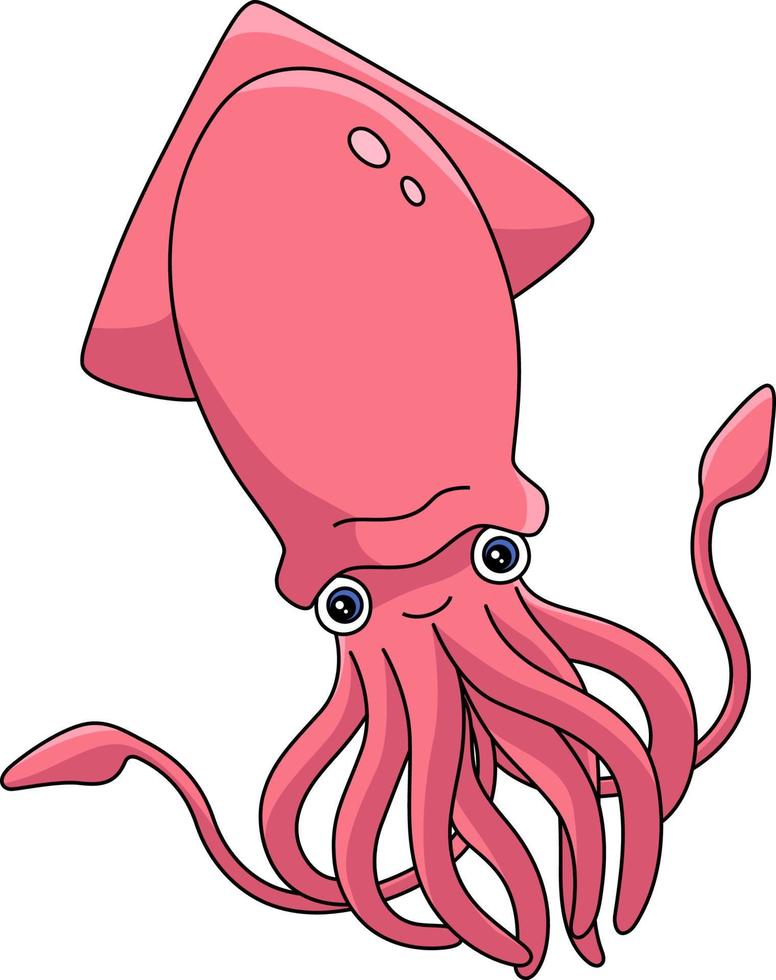This image is a cartoonish drawing of an octopus, predominantly in a reddish-pink or purplish-red color. The octopus features eight tentacles, with some spreading out to the sides and others dangling down. It has an elongated body that culminates in a nearly triangular shape at the top. There are two light spots on its head, enhancing its playful appearance. The octopus's eyes are white, accented with blue eyelids and a white glare, giving it an expressive look. Its cheerful smile is directed at the viewer, adding to its friendly and whimsical style, reminiscent of illustrations found in children's books. The background of the image is plain white, ensuring that the focus remains entirely on the lively and adorably drawn octopus.